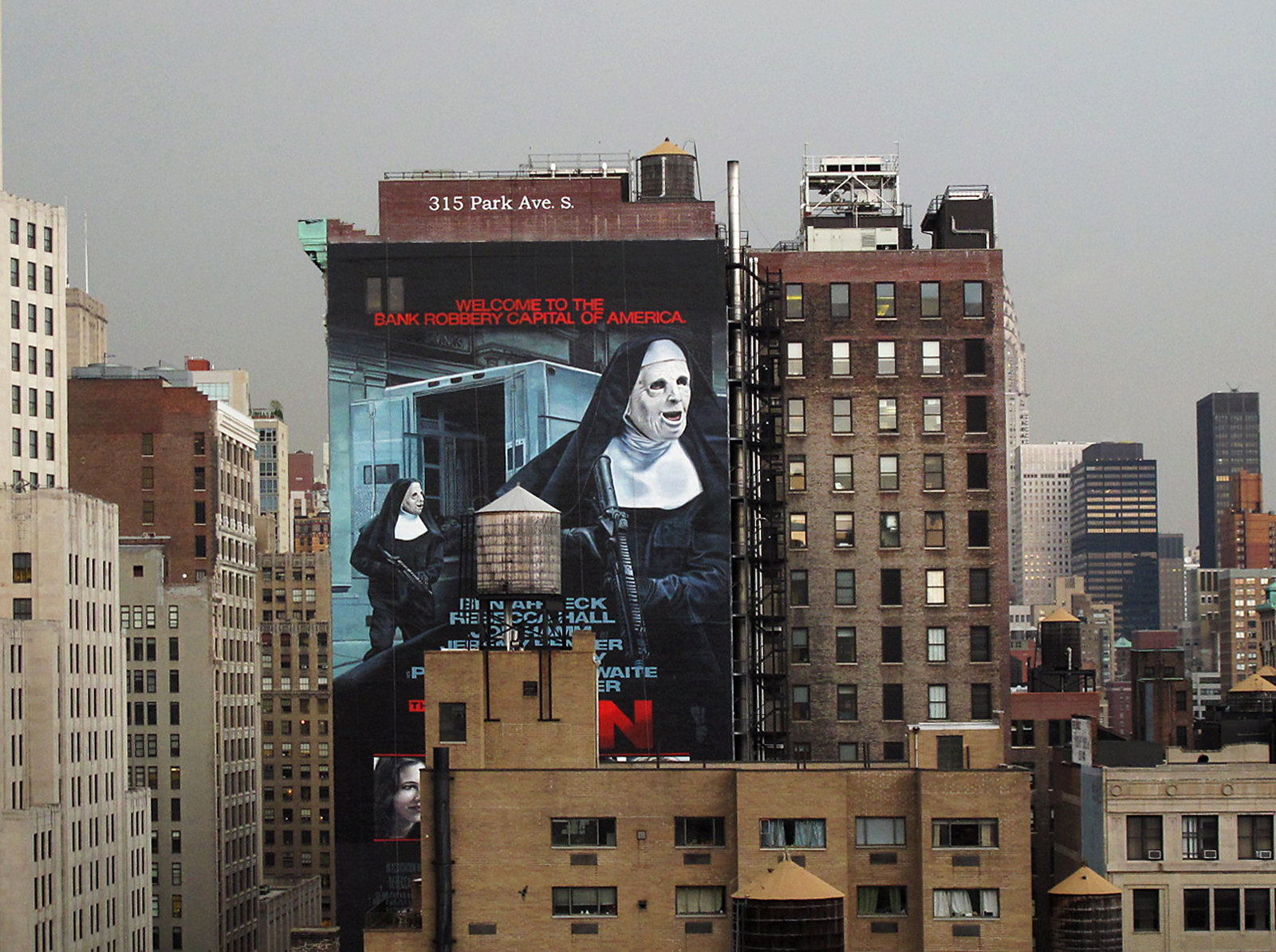The photograph captures a detailed city skyline under a flat, gray overcast sky. The diverse assortment of buildings extends from the older, red and gray brick structures and yellow-toned buildings in the foreground to the modern black and white skyscrapers in the distance. Dominating the scene is a red brick building with "315 Park Avenue South" clearly visible at its top, complete with a water tower, pipes, and rails. Prominently displayed on this building is a large billboard with a black background, promoting the movie "The Town." The poster features eerie figures in nun costumes with white masks, holding guns, seemingly emerging from a gray truck, and proclaims, "Welcome to the Bank Robbery Capital of America." The names listed, including a partially visible "Ben Affleck," are obscured by a nearby water tank and other structures. The city's architecture, ranging from classic apartment buildings with large windows and white curtains in various stages of openness to towering high-rises, paints a vivid urban landscape likely situated in New York City.